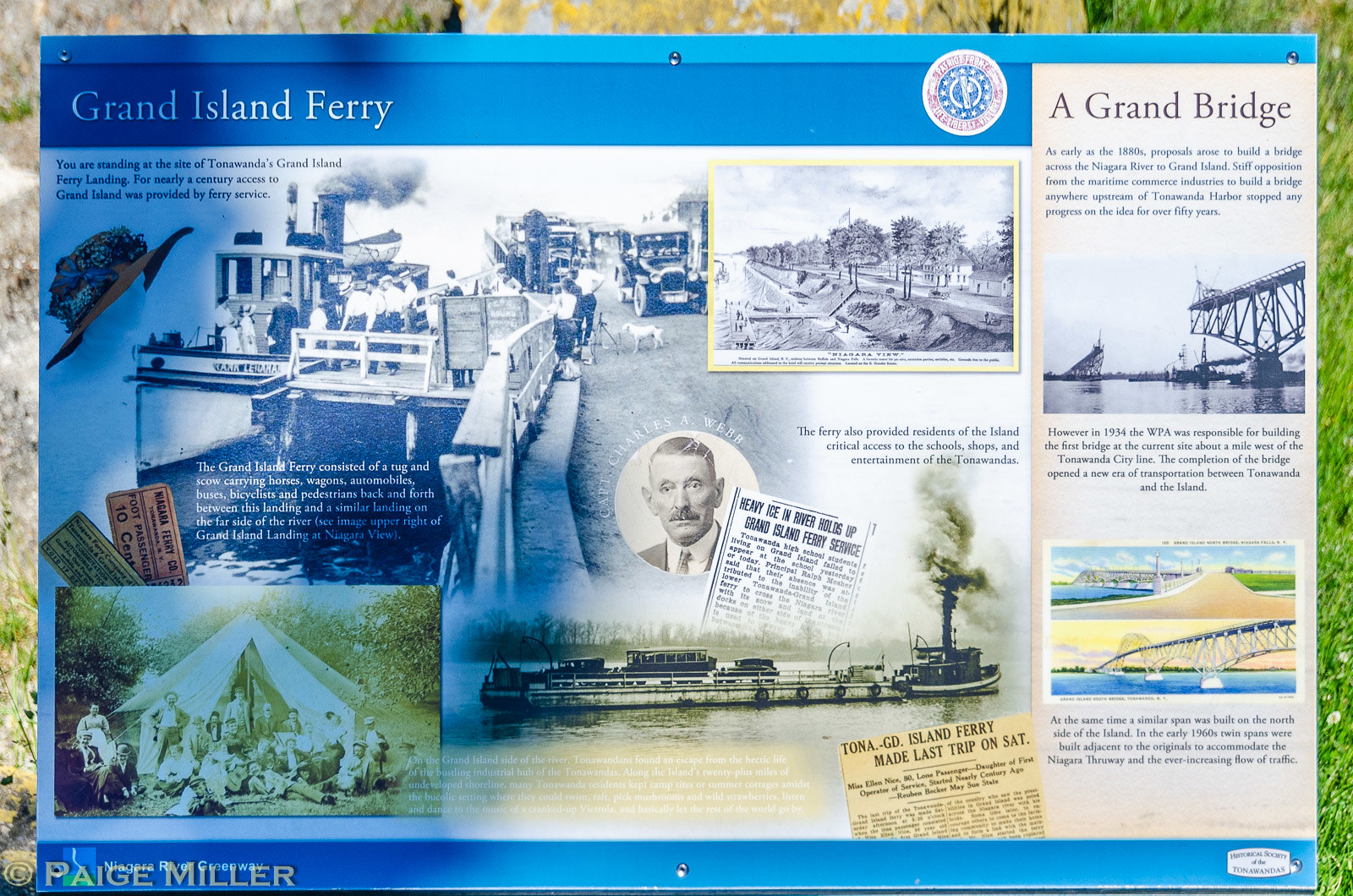This is an outdoor informational display with a blue and white design bordered by grass, stones, and rocks. Prominently labeled "Grand Island Ferry," the sign features multiple old-fashioned photographs and images. In the center, a black and white photo shows people boarding a small ferry from the early 1920s, with vintage cars and a dog nearby. Another image, tinted yellowy black and white, depicts a longer ferry accompanied by a small tugboat. There is a small inset photo of a mustachioed man in a suit holding a newspaper. On the right side of the sign, labeled "A Grand Bridge," you can see pictures related to the construction and completion of a bridge, including people camping outside a tent. The name "Paige Miller" is noted at the bottom left of the plaque.